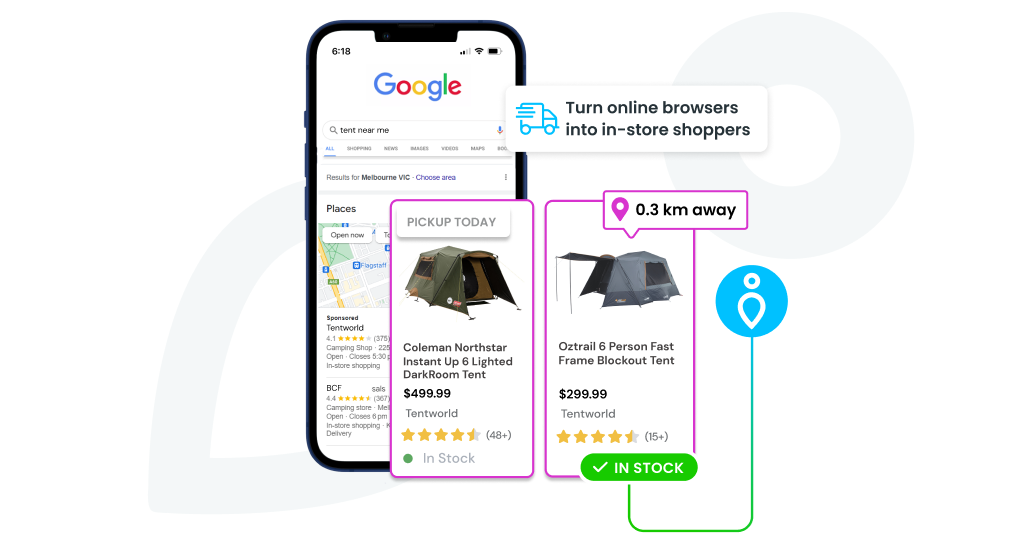The image is a screenshot displaying a Google Home search interface. The background is gray and features symbols, including a life preserver icon to the right and a heart tilted southwest behind the phone screen. The time on the device reads 6:18 A, though it doesn't specify AM or PM. The battery level is robust, estimated at around 80%. The word "Google" is prominently displayed at the top in its signature multicolored font.

The search query entered is "tent near me," and the device has produced various results. The search results are tailored to the address "Melbourne" and offer a feature to "choose area." Below, there are several search results that aren’t fully visible. Two entries are partially readable; one tent is rated 4 stars, another is 4.1 stars, and a third is 4.4 stars. The screen prominently displays the options to choose from:

1. **Coleman North Star Instant Up Tent** - Lighted dark room tent, 6 feet in height, priced at $499.99.
2. **Astrell Six-Person Tent** - Frame block out tent, priced at $299.00.

One of the visible tents is available at a store named "Trent World," located only 0.3 kilometers away, and the tent is confirmed to be in stock, ready for ordering.